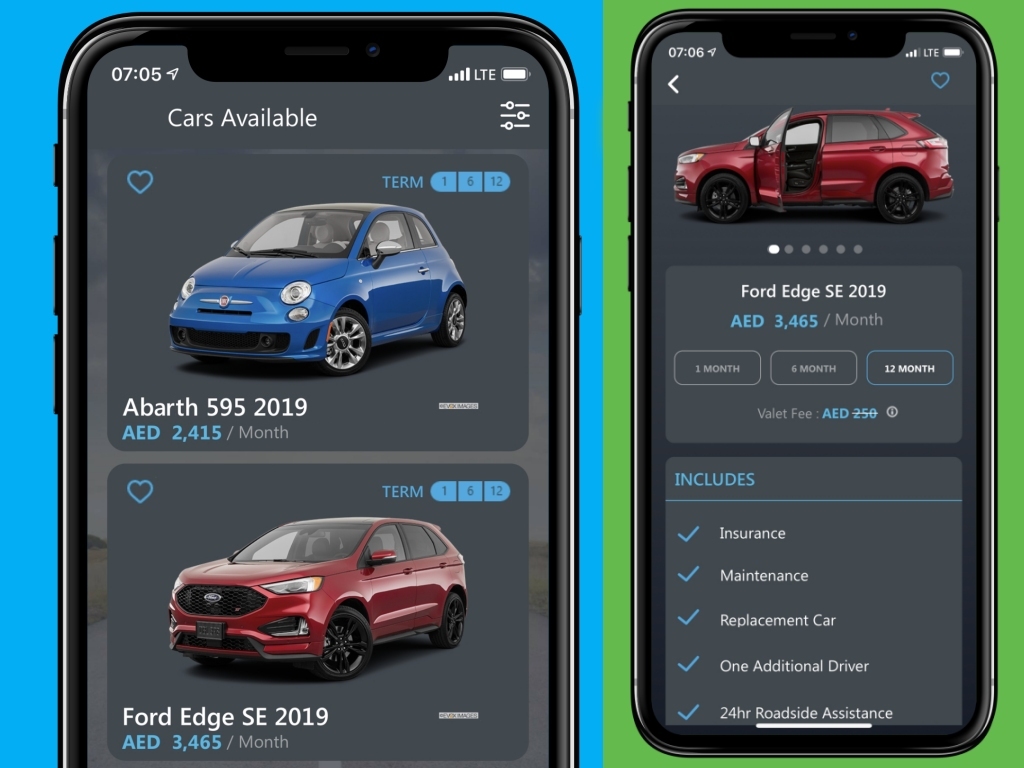Two smartphones are displayed side-by-side, both showing a car-selling website, although the exact site is not specified. The phone on the left features a blue background and displays key details, while the phone on the right has a green background with additional information.

On both screens, the time reads 7:05, and icons for LTE signal strength and battery life are visible at the top. The main page on the left phone shows the heading "Cars Available," indicating the availability of cars for sale. There is a heart symbol next to the heading for users to like or save the listing.

The first listing is for an Abarth 595 (2019) priced at AED 2,415 per month. This pricing is available across three different terms: 1 month, 6 months, and 12 months. 

The second listing is for a Ford Edge SE (2019) priced at AED 3,465 per month, also available for 1, 6, or 12 months. The user has clicked on this listing, which expanded to show more details.

Below the Ford Edge SE details, a valet service fee of AED 250 is mentioned. Additional features included in the price are insurance, maintenance, car replacement, one additional driver, and 24-hour roadside assistance.